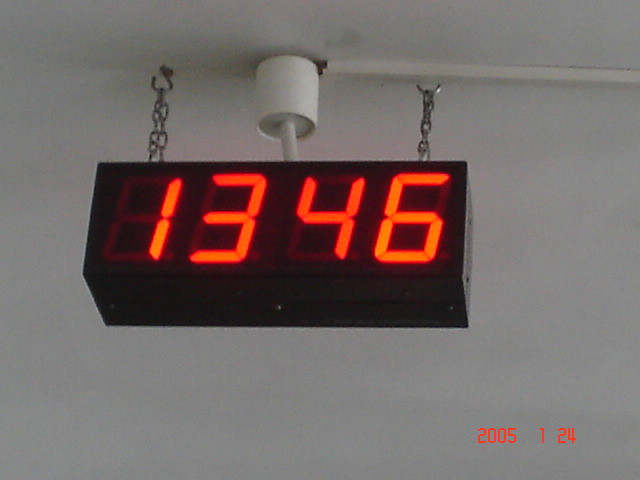In this photograph, dated January 24, 2005, a rectangular black digital clock with a red LED display hangs from the white ceiling by two silver chains attached to silver hooks. The clock reads "1346" with segments of the numbers visible in an unlit state. Behind the clock, a cylindrical white electrical duct with a white rod can be seen, providing power to the clock. The white ceiling and wall serve as a stark contrast to the black housing of the clock, making it the focal point of the image.